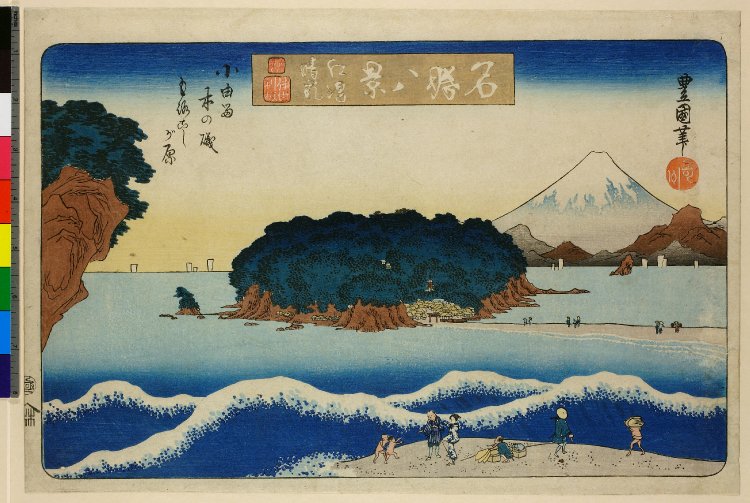The image is a detailed, rectangular Japanese poster reminiscent of an old postcard, approximately six inches wide and three inches tall. It features a beige banner across the top with white Japanese characters and black calligraphy on the left and right sides, alongside red stamps. Dominating the center is a small, verdant island with dark green treetops and brown trunks, surrounded by a light blue ocean that transitions to darker blue with white-capped waves in the foreground. A beige path leads to the island, dotted with people walking. The scene includes a sandy beach in the foreground, also populated with people and children. In the distant right background, the majestic, snow-capped Mount Fuji rises, flanked by additional brown and gray mountains. The sky above showcases a gradient of blue, white, and yellow hues, completing the serene and picturesque setting.